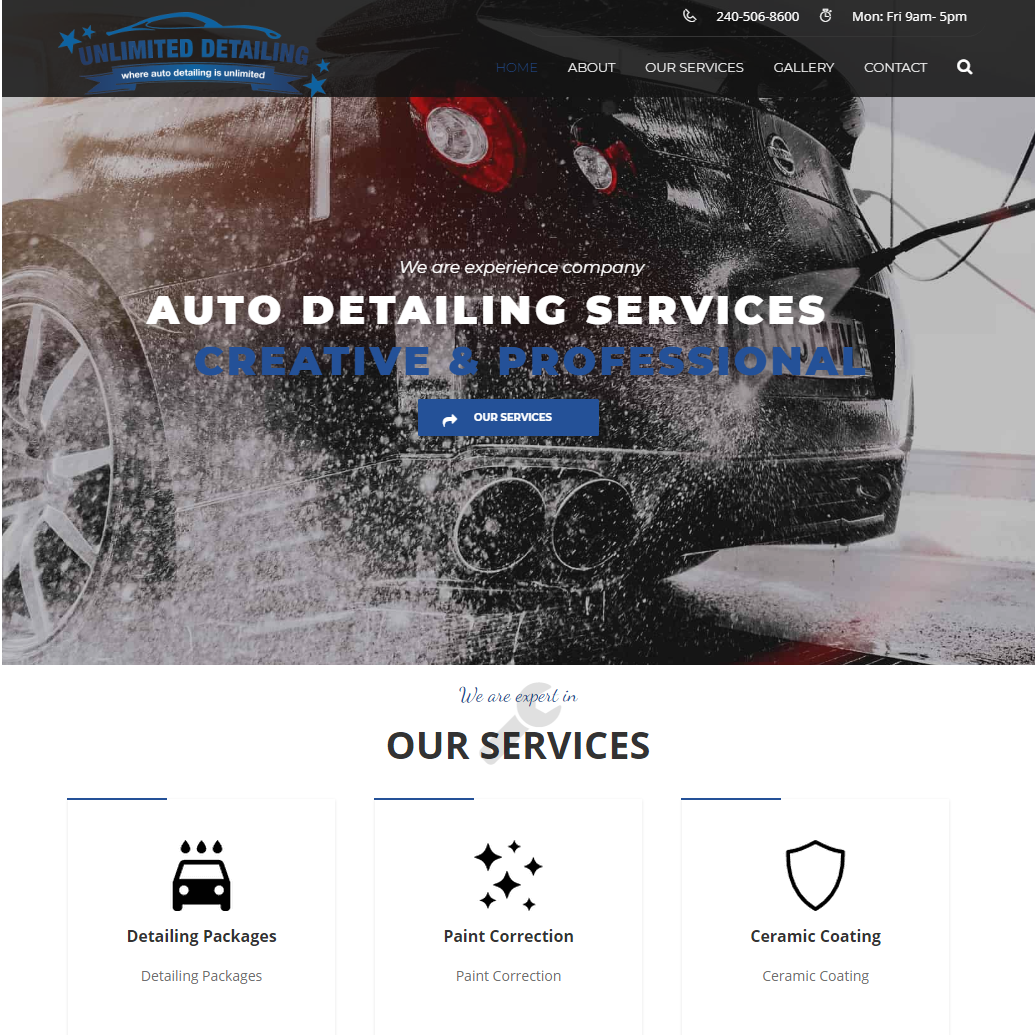This website, Unlimited Detailing, showcases their comprehensive auto detailing services. In the upper left corner, the site name "Unlimited Detailing" is prominently displayed. To the right, starting in the middle, there are navigation links labeled "About," "Our Services," "Gallery," "Contact," and an icon for search functionality. Above these links, the company's phone number, 240-506-8600, and business hours, Monday through Friday 9 a.m. to 5 p.m., are positioned clearly.

Dominating the webpage is a striking photograph of the rear end of a sleek black car, likely a Nissan, complete with European license plates. The red brake lights are illuminated, and water is seen splashing up around the vehicle, adding a dynamic effect. Superimposed over the image, in bold lettering, the caption reads "Auto Detailing Services - Creative and Professional." Below this, a blue button with white text invites visitors to explore "Our Services."

Above the primary tagline, in smaller text, the site claims "We are an Experienced Company," indicating their proficiency in the field, although the phrasing is somewhat awkward. Beneath the main image, on a white background, additional services are listed, including "Detailing Packages, Paint Correction, and Ceramic Coating."

The website features a color scheme of blue, black, white, red, silver, and gray, creating a sleek and professional aesthetic.